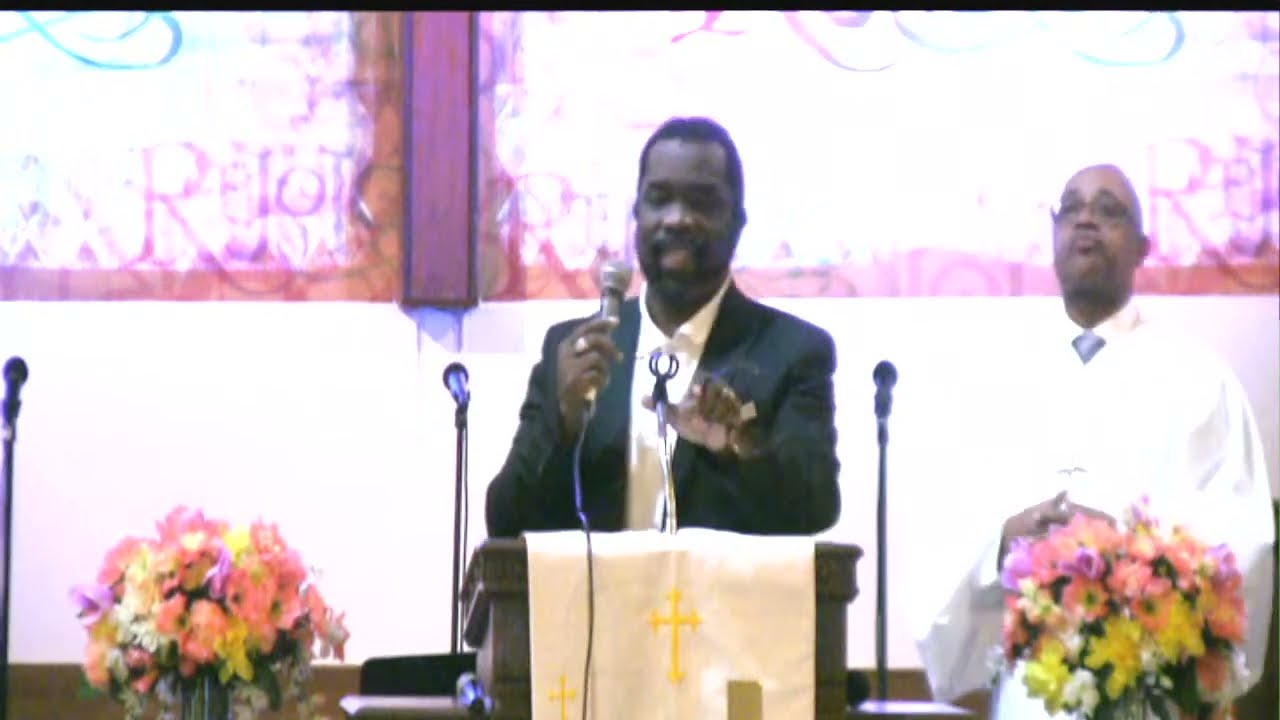In this detailed image set in what appears to be a church in the middle of the day, we see two African American men positioned prominently. At the center, a man with a beard and mustache, wearing a black jacket over a white polo shirt, stands at a podium adorned with a white cloth featuring gold crosses. He is actively speaking, holding a corded microphone in his right hand and gesturing with his left hand. To his right, another man dressed in a white choir or minister's robe with a blue necktie is standing in front of a floral arrangement, seemingly looking upwards and wearing glasses. Both men are dressed formally and contribute to the atmosphere of a religious service. Flanking the podium are two bouquets of flowers in shades of pink, peach, lavender, yellow, and white. The background features stenciled decorations on the walls, adding to the church setting. Bright light filters in, enhancing the colorful and reverent ambiance of the scene.